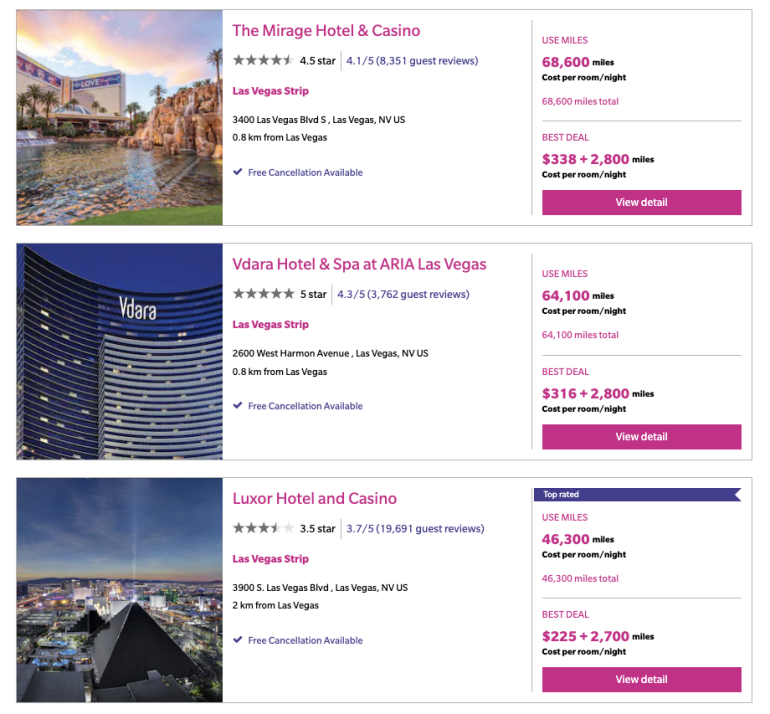This detailed caption should fit your request:

"On this hotel booking website, a vertical list features three prominent hotels in Las Vegas, displayed from top to bottom. Each entry consists of key visual and informational elements. On the left, a photograph showcases the exterior of the hotel: the Mirage Hotel is listed first, followed by the Vidara Hotel, and finally the Luxor Hotel. Adjacent to each image is a detailed description box.

The box provides the hotel's name and star rating at the top, followed by the number of guest reviews and their average rating out of five. Next, the location is specified as the Las Vegas Strip, with the hotel's complete address in black text beneath it. An additional note mentions that free cancellation is available.

To the far right of each entry, two sections offer booking options. The first option allows guests to use 68,600 miles per night, while the second presents a 'best deal' that combines $338 plus 2,800 miles per night. To conclude, a pinkish button labeled 'View Details' encourages users to explore more information about each hotel room."